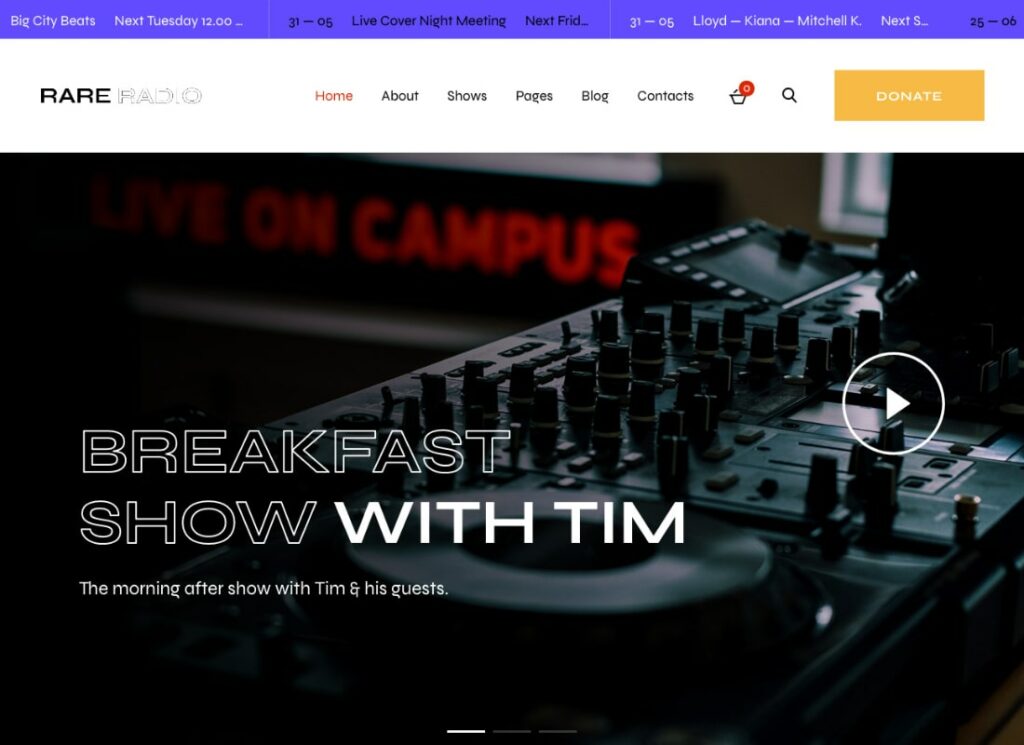The image showcases a dark background that serves as a holding page for an unspecified video, denoted by a play symbol. Embedded within this background is subtle, red text reading "on campus," suggesting a connection to campus events. In the foreground, there is an image reminiscent of a mixing board, hinting at a broadcast or audio production theme.

Dominating the center is prominent text announcing "Breakfast Show," outlined in white with hollow letters, and "with Tim" in bold, solid white, emphasizing Tim's role as the host. Beneath, it reads, "The Morning After Show with Tim and his guests," suggesting a follow-up discussion about recent campus happenings.

At the top, a blue banner with small, hard-to-read text mentions "Big City Beats" and other details seemingly related to a Tuesday event at 12 o'clock. This is followed by various, partially obscured listings such as "live cover night" and names like "Lloyd," "Chiara," and "Mitchell."

The navigation bar below includes options such as Home, About, Shows, Pages, Blog, Contest, Contacts, and a shopping cart icon. Additionally, there's a search option and a prominent "Donate" button.

The combination of these elements suggests a dynamic and interactive platform, possibly a radio station or a media site named "Rare Radio," facilitating various shows and events.